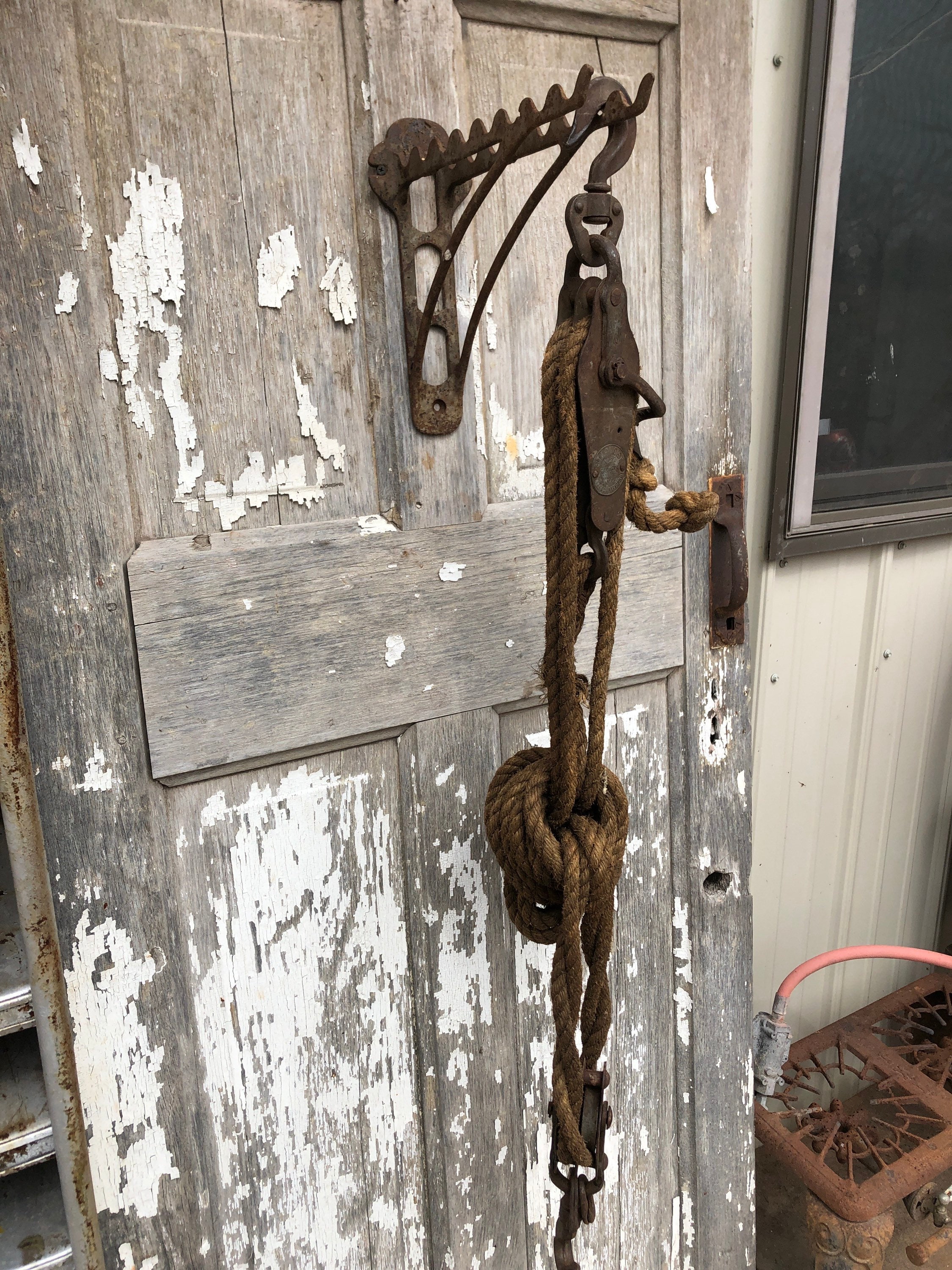The photograph is an outdoor scene showcasing a strikingly rustic setting. The focal point is an old, weathered wood door, originally painted white but now mostly chipped away, revealing a grayish-brown wood beneath. This door, no longer on its hinges, leans against a white sheet metal building, exuding a distinctly shed-like appearance. A rusted metal bracket adorns the top of the door, equipped with a hook and a pulley system with a dangling brown rope, hinting at its past utilitarian purpose. To the right of the door, a brown-framed screen window offers a glimpse of the building's interior. Below the window sits a rusted brown bench, likely made from cast iron or a similar metal. Additional elements, such as upside-down baskets, one with a peach-colored drawstring, add to the scene’s authenticity and charm, embodying a sense of timeworn simplicity.